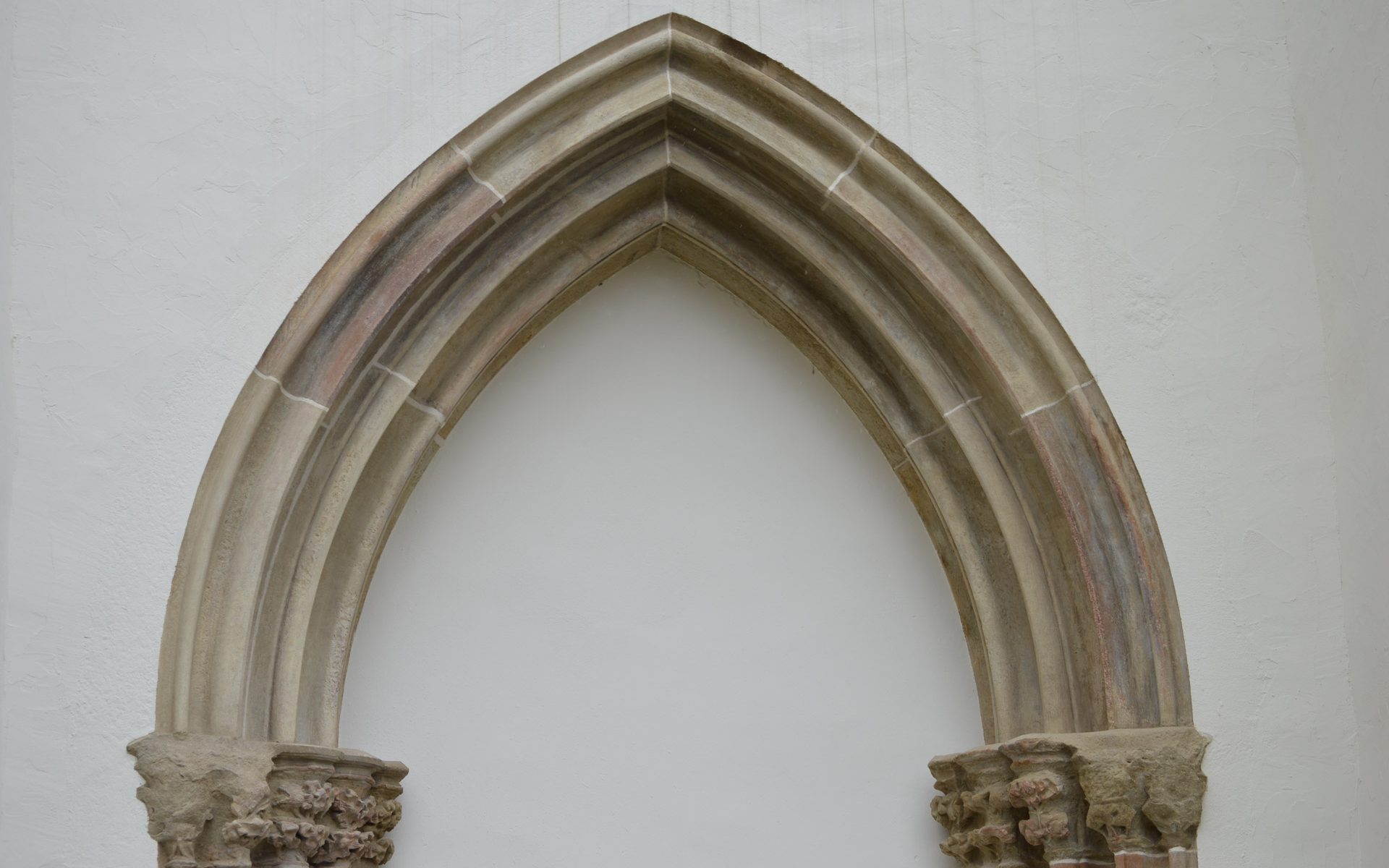The image showcases a stone archway set against a white or light gray background, reminiscent of a museum display. The arch itself is distinctively triangular at its peak, distinguishing it from the more common rounded arches. Composed of a light sandstone color with darker brownish-gray highlights indicating ridges, the arch exhibits subtle textures and natural stone variations. The legs of the arch extend down into two wider columns at the base, which feature minimalistic carving to accentuate their shape. These columns appear somewhat eroded by time, adding a sense of historical depth. Grooved channel-like sections, resembling stairs, ascend from the flat platforms at the base of each column, emphasizing the arch's structural intricacy. Though the exact historical style of the columns is unclear, their worn appearance contributes to the archway's ancient and timeless aesthetic.